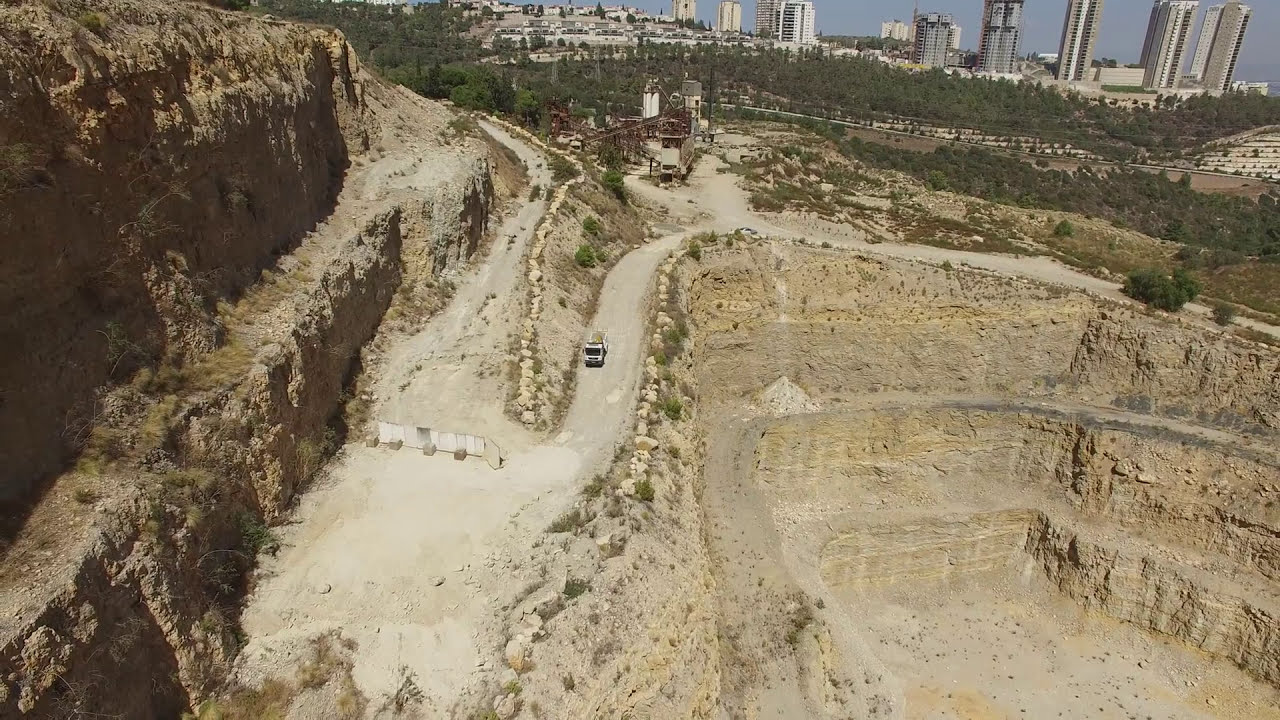An aerial view reveals a vast rock quarry embedded within a hill or mountain, characterized by extensive rocky and stone-filled landscapes composed of brown, tan, and black hues, interspersed with patches of green grass and vegetation. The scene is dominated by vertical rock bluffs and dirt cliffs, creating a rugged and industrial aesthetic. A winding dirt road, carved meticulously into the stone, descends into the quarry's depths, upon which a large dump truck is visible, navigating toward an opening fortified by a white barricade held up by stones. Surrounding the quarry is a network of dirt roads. In the background, a small metropolitan area punctuates the horizon, featuring a blend of gray one-story residential homes and approximately ten tall commercial buildings and white skyscrapers. The metropolitan skyline is encircled by dense forestry, with a mix of green trees stretching across the landscape, enhancing the contrast between the barren quarry and the verdant city outskirts.